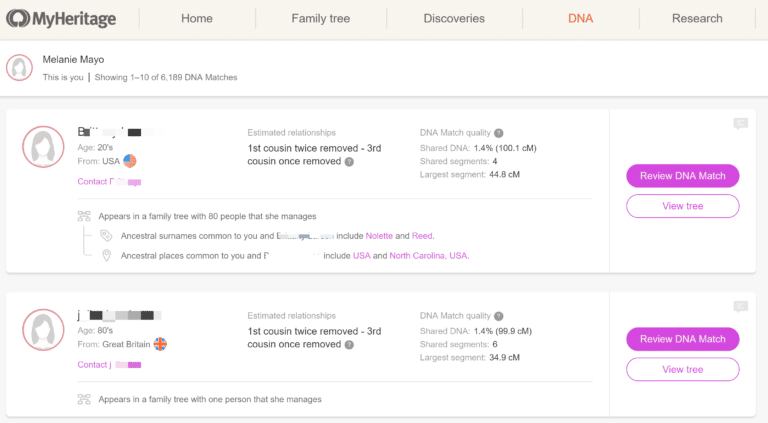The screen capture features the interface of the MyHeritage application. At the top left, the MyHeritage logo is prominently displayed. The header is a light tan color and includes a navigation bar with the following options separated by vertical bars: "MyHeritage" on the far left, followed by "Home," "Family Tree," "Discoveries," "DNA" (highlighted in red, indicating the current menu), and "Research." 

Below the navigation bar, a user profile section features a small red circle containing a girl's face and the name "Melanie Mayo," with a label indicating this is the user's profile. The caption informs Melanie that she is viewing "1-10 of 6,189 DNA matches."

Beneath this information is a gray box containing two white boxes. The first box has some information blanked out, but it indicates an individual in their 20s from the USA. Contact details are also redacted. The estimated relationship to Melanie ranges from "first cousin twice removed" to "third cousin once removed." Additional genetic details include a shared DNA percentage of 1.4%, four shared segments, and the largest segment measuring 44.8 cM. Further specifics continue in the document.